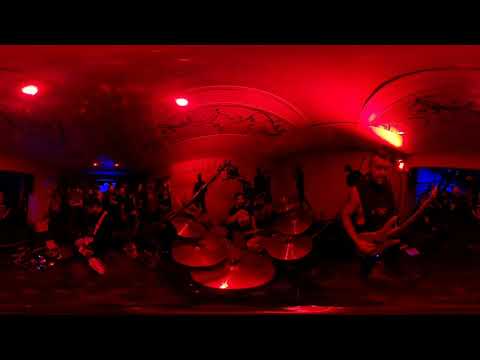The image is a color photograph taken inside a nightclub, predominantly lit in a brilliant red haze, producing a very dark and moody atmosphere. It appears to be a still shot, possibly taken with a fisheye lens and combined with a panoramic filter, resulting in a striking, wide-angle view. The photograph shows a band on a small stage, which spans the horizontal center of the image.

In the composition, a guitarist wearing a black tank top is positioned on the right, holding an electric guitar. On the left, a drummer is visible behind his cymbals. Toward the center background, potentially the lead singer, another person is standing. There are a few more indistinct figures in the background, barely visible due to the dim lighting.

The ceiling, also illuminated in red, features three overhead lights—one in the top left corner, another towards the left but centered, and a third light towards the right. Alongside the red ambiance, splashes of orange, royal blue, yellow, black, and white are present, adding to the vibrant but dark aesthetic of the nightclub setting. There are blue screens flanking the guitarist and drummer, enhancing the scene's surreal, immersive quality. The photograph is cropped with black horizontal strips at the top and bottom, further emphasizing the wide-angle, panoramic view of this dynamic live performance.